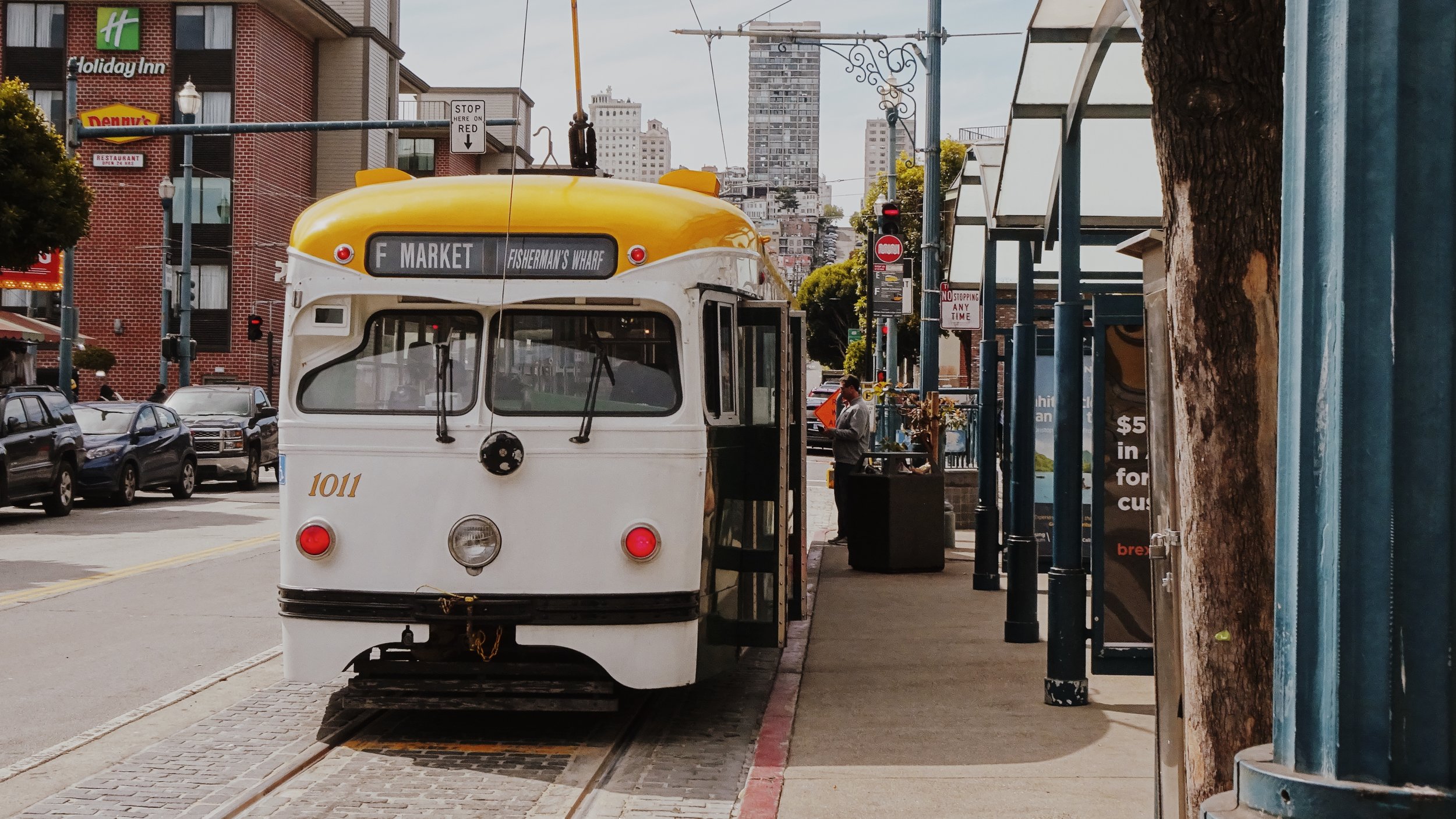In this detailed image taken outdoors during the daytime in a bustling city, the main focus is a white streetcar with a distinctive yellow roof, marked with the number 1011. The streetcar, which is part of the F Market & Fisherman's Wharf line, displays two red lights and a central white light at the front. It is hooked up to the railings embedded in a brick road and has its doors open. To the right of the streetcar, there is a sidewalk bustling with pedestrians and a bus stop station featuring green poles and white shelters. In the background, various buildings are visible, including a four to five-story Holiday Inn and a Denny's, both situated on a brick building. Further in the distance, the city skyline with skyscrapers stretches across the horizon. The scene is complemented by clear weather with minimal clouds, ensuring excellent visibility of the urban landscape. Traffic lights and typical city traffic add to the lively environment.